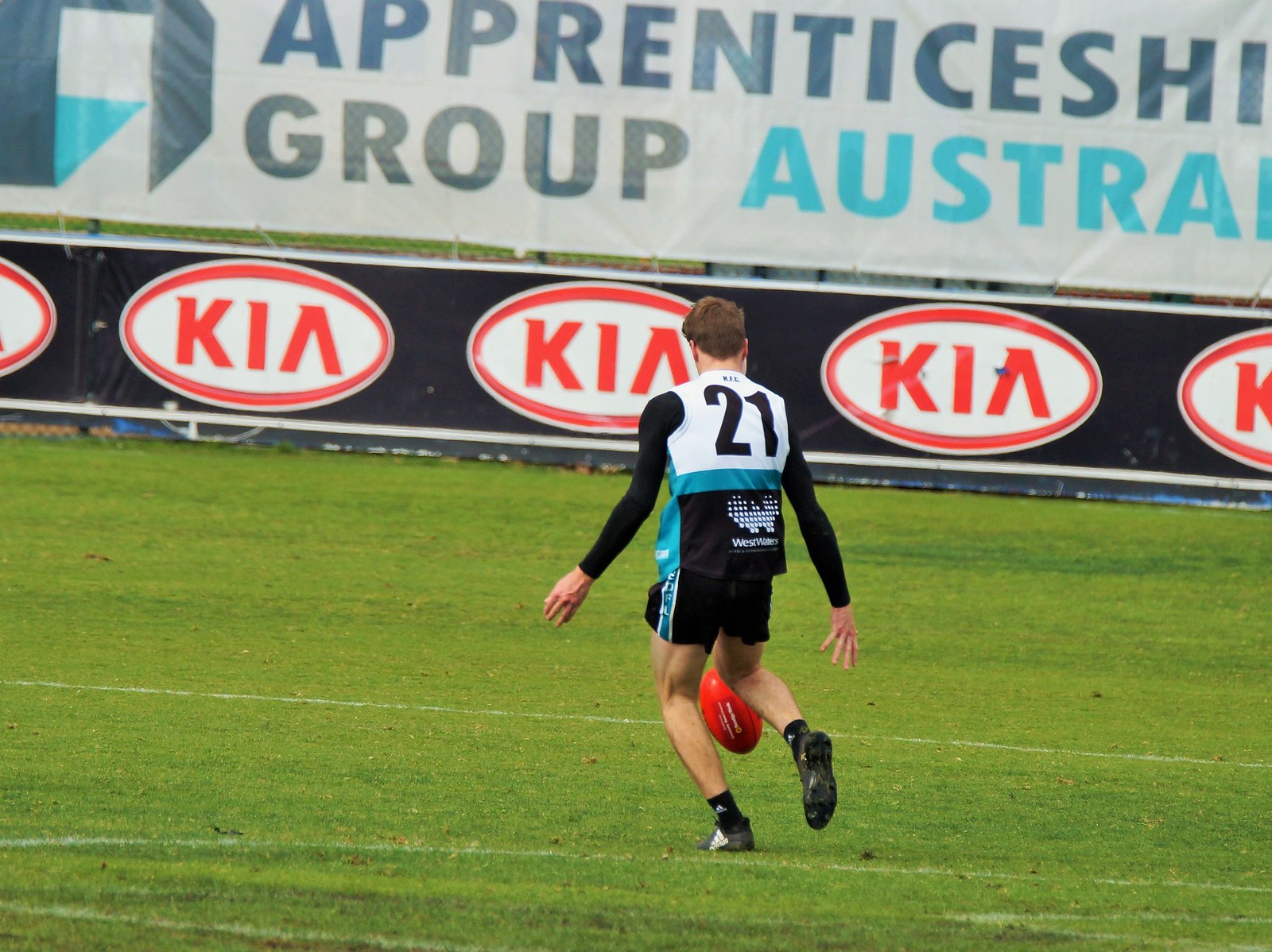The photograph captures a moment during an outdoor sports event on a green field, featuring a man in motion. He appears to be a soccer player but is actually engaged in kicking a red football, which is uncharacteristic given the oval shape of the ball, typically used in American football or rugby. Notably, he is not wearing the traditional heavy padding and helmet associated with American football; instead, he dons standard soccer attire, including regular shorts, a jersey, and a black long-sleeved shirt underneath the jersey. His outfit includes dark trunks with a blue band on the side, dark socks, and reddish shoes, suggesting it is quite chilly as he is dressed warmly. The backdrop features various advertisements, prominently displaying a banner reading "Kia" against a black and blue background, as well as signage for "Apprenticeship Group Australia". The overall scene conveys a collision of sports traditions, heightened by the unusual choice of attire and equipment for the activity depicted.